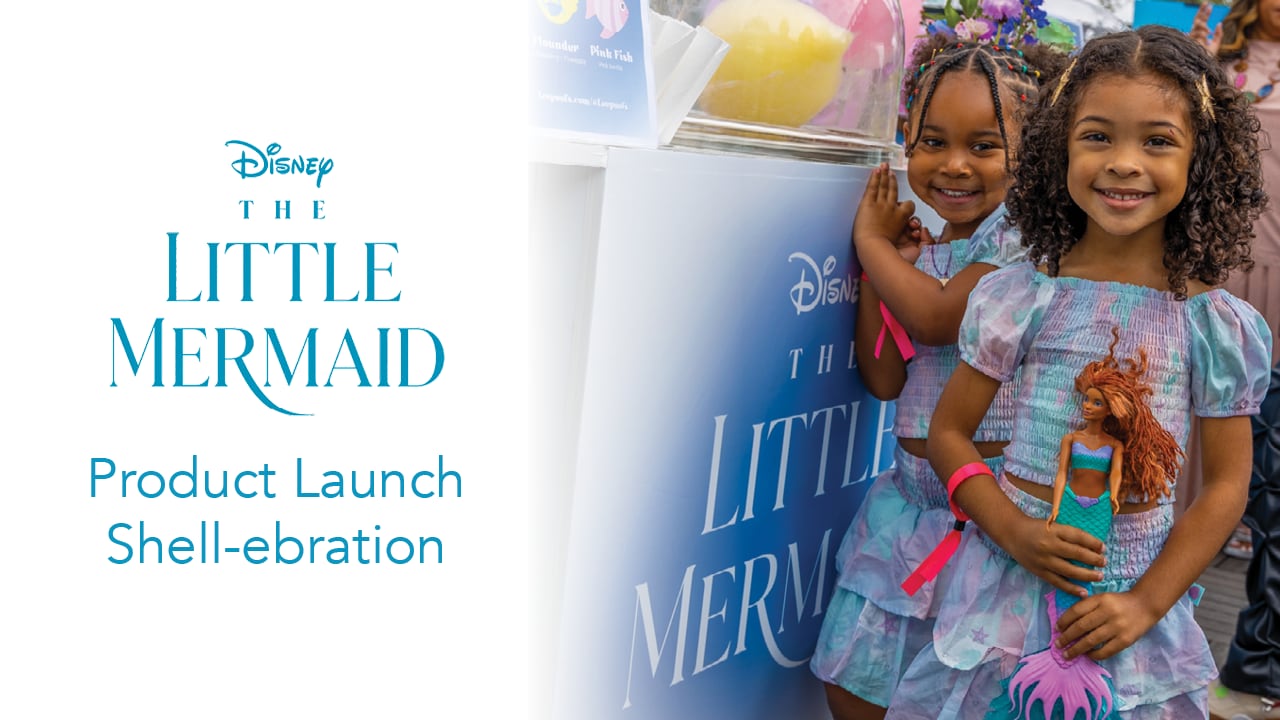In the image, there are two young African-American girls standing on the right side, smiling joyfully in front of a "Disney The Little Mermaid" poster at a product launch celebration. Both girls have dark hair, with the one in the back sporting an updo and the one in front wearing her hair down, adorned with two hair bow barrettes on each side. Their outfits are matching two-piece sets consisting of a shirt and a skirt with puff sleeves and ruching, in a multicolored palette of blue, purple, green, and pink tie-dye that mirrors the colors associated with Ariel, the mermaid. Each girl has a hot pink wristband, possibly serving as an identifier for the event. The girl in the front is holding a doll resembling the new black Little Mermaid, dressed in a greenish-blue top and fin with a pink tail. The left side of the image features a white background with blue text that reads, "Disney The Little Mermaid Product Launch Celebration." Behind the girls, there are various colors and possibly other people, contributing to the lively atmosphere of the event.